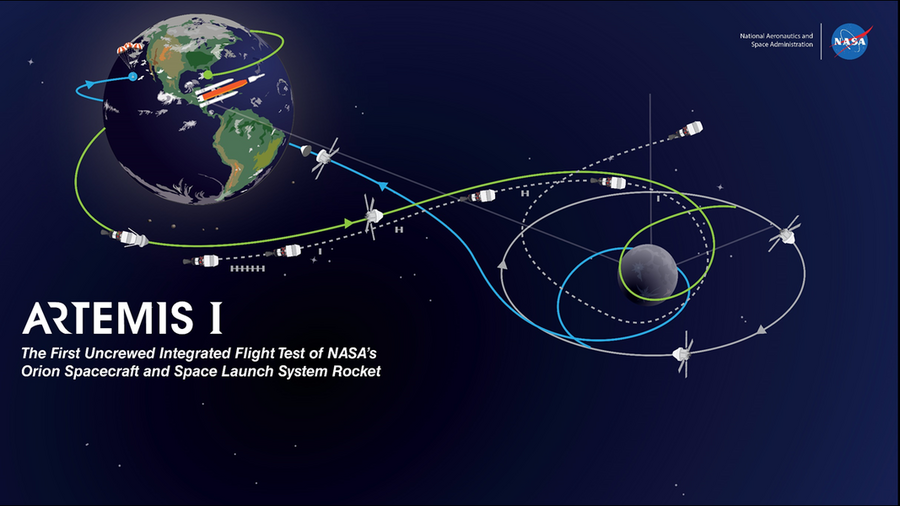This detailed cartoon diagram depicts the Artemis 1 mission, the first uncrewed integrated flight test of NASA's Orion spacecraft and Space Launch System (SLS) rocket. The background is a gradient of deep blue and black, speckled with white dots representing stars. In the lower left corner, white text reads: "Artemis 1, the first uncrewed integrated flight test of NASA's Orion spacecraft and Space Launch System rocket." The image’s focal point is a cartoon render of the Earth on the left, featuring an orange spaceship with its solid rocket boosters. A green line trails from the spaceship, illustrating its orbital trajectory as it wraps around the Earth and heads towards the moon on the right. As the trajectory nears the moon, the line transitions from green to blue, showing the spacecraft's return path as it loops around the moon and heads back towards Earth. The spacecraft is shown in various mission stages, including solar panel deployment and re-entry preparation, culminating in a depiction of its landing in the ocean. The top right corner of the image features the NASA logo with the accompanying text "National Aeronautical and Space Administration." The visual succinctly captures the mission's journey through space and its significant stages, serving as an educational tool for understanding this pioneering flight test.